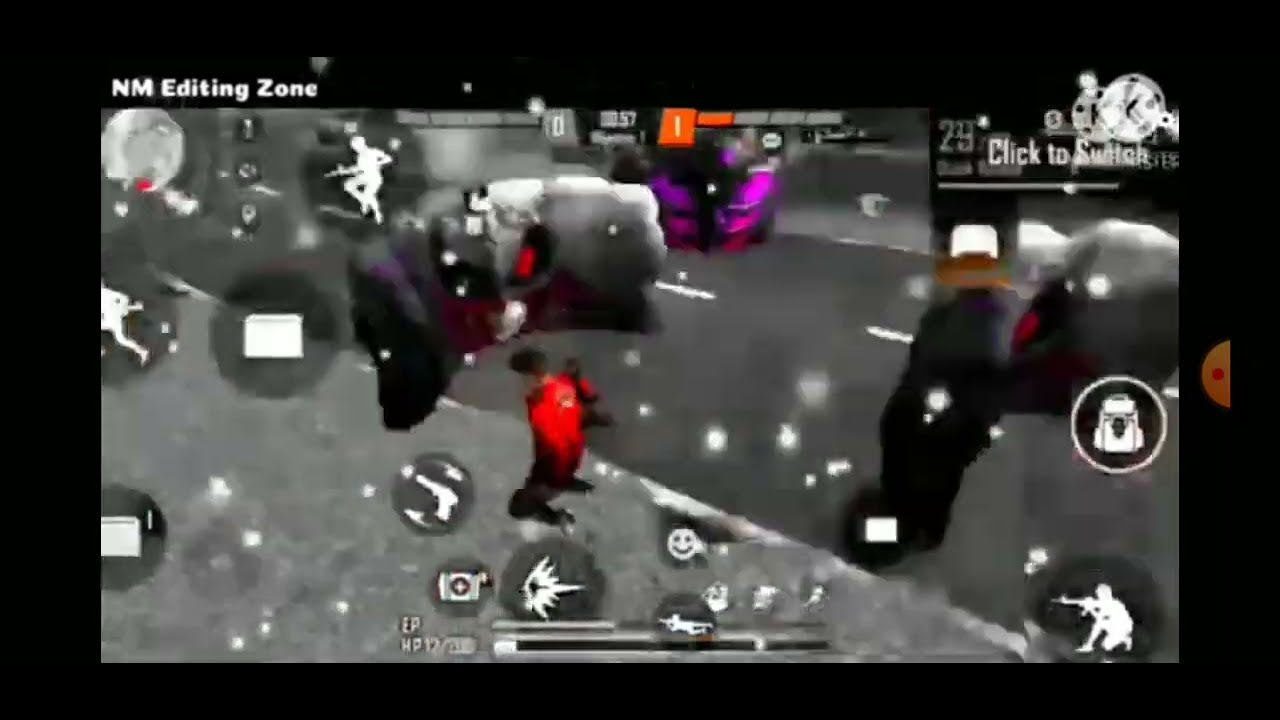This screen grab from a blurry and poor-quality video game scene features a black background with a gray street running diagonally from the bottom right to the top left, marked with white passing lanes. The central focus is a red creature with black feet, its exact details unclear due to the image's blurriness. Above this creature is an indeterminate gray figure with striking features including white teeth and red eyes. Behind this is another black object with purple spots. The scene also includes numerous icons, potentially representing soldiers, smiley faces, explosions, and guns, possibly indicating a menu or interface screen. In the lower right and upper left corners, there are white silhouette figures in shooter's poses; one appears to be kneeling with an assault rifle, and the other seems to be jabbing with a bayonet. Text overlays are present including "NM editing zone" in the top left corner, and "click to switch" in the top right. Additionally, a health point bar is visible at the bottom, accompanied by an orange bar graph at the top center with four bars, where only the first bar is orange and the others are dark gray. The game's general imagery is predominantly grayscale, with occasional pops of red and purple, contributing to a chaotic and action-filled atmosphere.